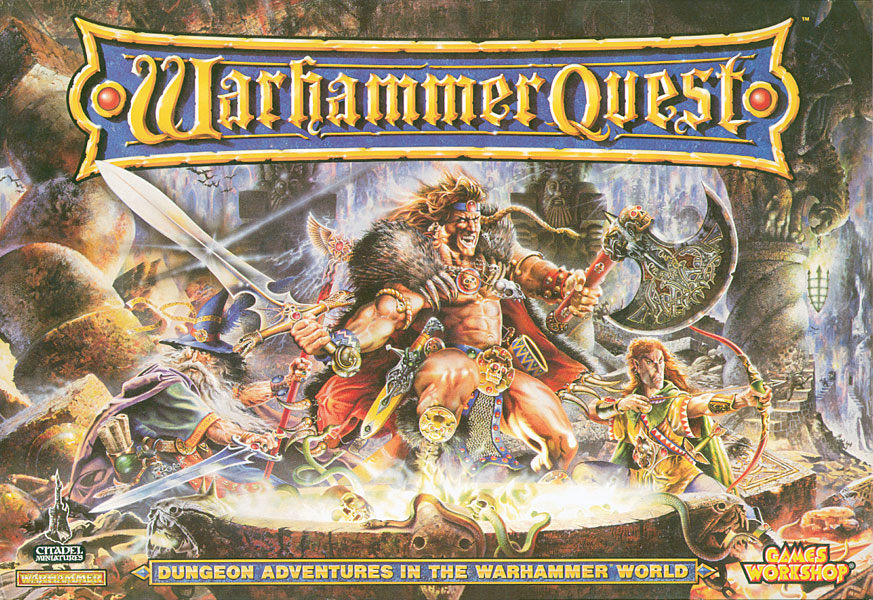The image is a horizontally aligned rectangular cover for the board game "Warhammer Quest" featuring an elaborate and dynamic central design. Dominating the center is a bare-chested, muscular warrior with long, wavy brown hair tied back by a blue and red bandana. He appears to be in the midst of battle, screaming with his mouth wide open. In his right hand, he wields a shining sword with a bright white blade, while in his left hand, he holds a weapon with a red handle, possibly an axe. He is adorned with a red cape and brown fur around his neck and head, and his legs are bare except for something wrapped around his waist and kneecaps.

Flanking the central warrior are two additional characters: to his lower right, an elf archer is poised with a bow and arrow, wearing some form of gown; to his left stands a wizard dressed in a gown and wizard hat, brandishing a staff. They appear to be in a dungeon, standing behind what looks like a cauldron filled with skeletons and snakes, with light emanating from below them.

The game title "Warhammer Quest" is prominently displayed at the top of the cover in gold letters with a medieval font, set against a blue background with gold trim and red rivets at each end. At the bottom of the cover, the subtitle "Dungeon Adventures in the Warhammer World" is written in yellow letters on a similarly designed blue and gold banner. The name "Games Workshop" is also featured in the lower right corner in gold letters. The art conveys a sense of epic fantasy adventure, characteristic of the Warhammer universe.